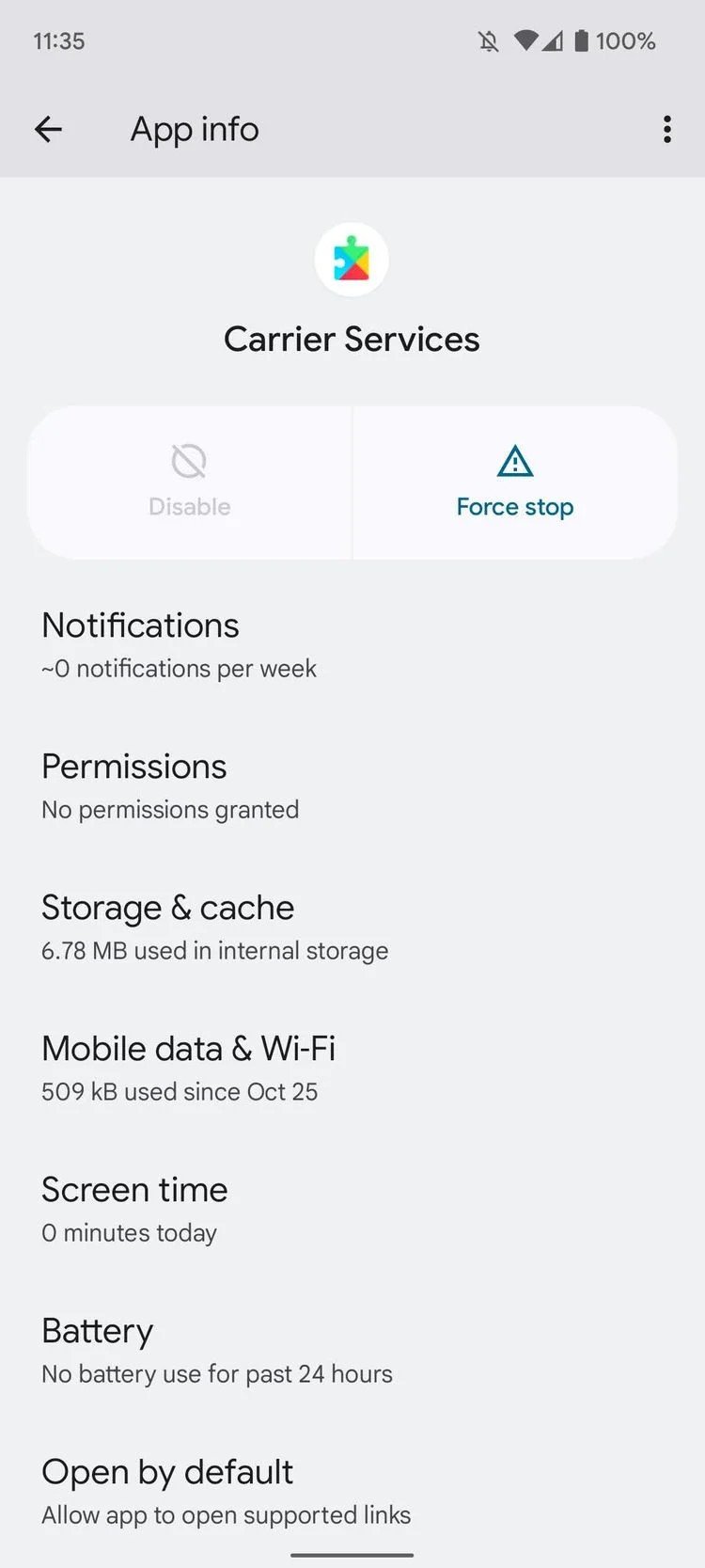The image depicts a long, vertical rectangle with a predominantly gray backdrop, divided into distinct sections resembling a smartphone screen interface.

At the very top, a darker gray rectangle features standard phone screen indicators. On the left, the time is displayed as 11:35. To the right, a series of icons can be seen: a crossed-out bell indicating silent mode, a full Wi-Fi signal depicted as a rounded triangle, three vertically ascending bars with the third bar hollow, and a full battery icon with "100%" beside it. Below this status bar, the words "App Info" are centered, flanked by a left-pointing arrow on the left and three vertical dots on the right.

The section below this is a lighter gray rectangle. Centered at the top is a white circle containing a multi-colored puzzle piece with green at the top, blue on the left, yellow on the right, and red on the bottom. Next to the puzzle piece, it says "Carrier Services."

Below this, there is a light gray, rounded rectangle divided into two parts. On the left, the word "Disable" is accompanied by a circle with a cross above it. On the right, "Force Stop" is written in turquoise with a triangular warning icon above it.

The interface continues with various headings and corresponding information, each section starting with bold, larger font:
1. **Notifications:** Below it, a squiggly line and "0 notifications per week," in a smaller, less bold font.
2. **Permissions:** Below it, "No Permissions Granted," in a smaller, less bold font.
3. **Storage and Cache:** Below it, "6.78 MB used in internal storage," in smaller, less bold font.
4. **Mobile Data and Wi-Fi:** Below it, "509 KB used since Oct 25th," in smaller, less bold font.
5. **Screen Time:** Below it, "0 Minutes Today," in smaller, less bold font.
6. **Battery:** Below it, "No Battery Use for the Past 24 Hours," in smaller, less bold font.
7. **Open by Default:** Below it, "Allow App to Open Supported Links," in smaller, less bold font.

At the very bottom, a thin horizontal rectangle is centrally located, with ample space on either side.

This detailed description captures the functional layout and specific information displayed in the image, effectively communicating the organized and informative nature of the smartphone interface.